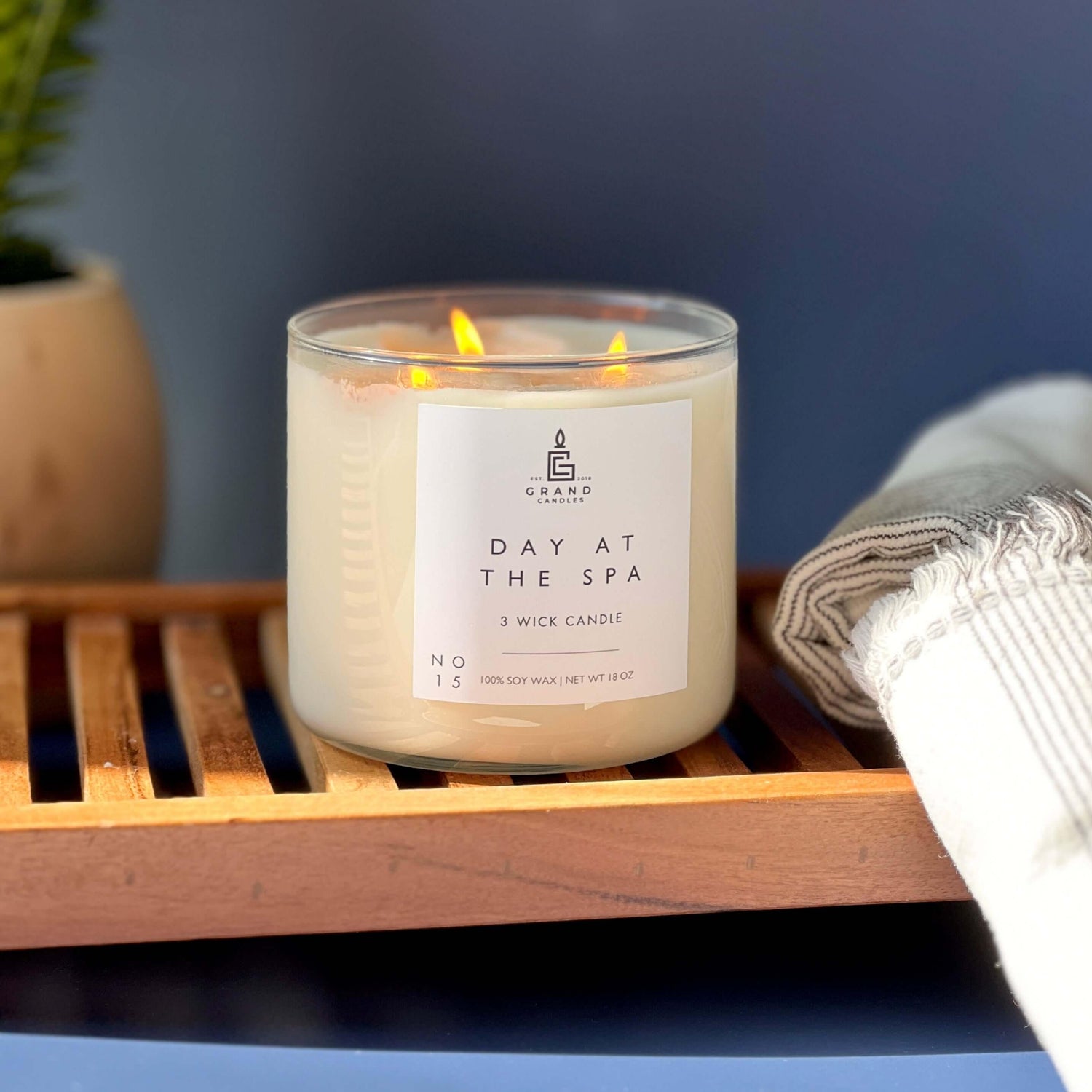The image depicts a serene spa scene with a dark blue wall in the background. On the left side, a tan pot with green leaves peeks into the frame. The focal point of the photo is a glass jar candle, which is creamy white in color with three lit wicks emitting small flames. The candle rests on a wooden slatted tray, resembling a small pallet. The candle's label, set against a white background with black lettering, reads: "Grand Candles, Day at the Spa, Three Wick Candle, Number 15, 100% Soy Wax, Net Weight 16 ounces." 

Adjacent to the candle on the wooden tray is a fluffy, rolled-up towel, either white or striped with gray. Another towel, partially rolled, balances next to the tray. The overall setting exudes a calm, spa-like atmosphere, enhanced by the soft candlelight and the organized arrangement of spa accessories.